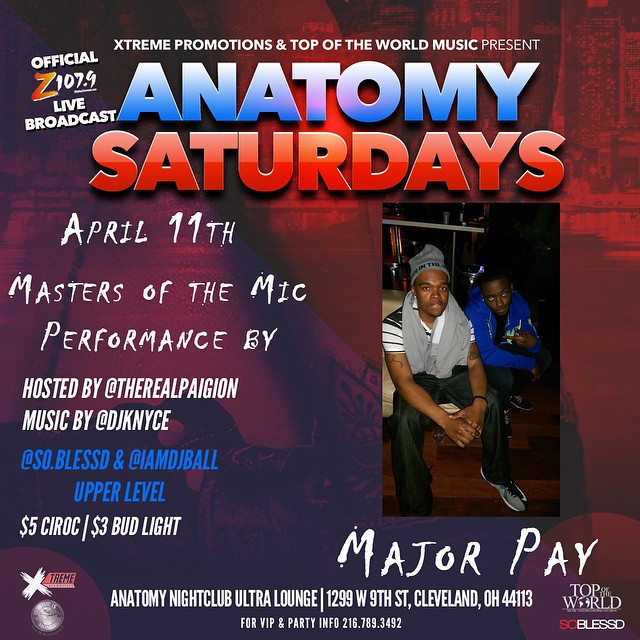This vividly-designed advertisement promotes an event at Anatomy Nightclub, located at 1299 West 9th Street, Cleveland, Ohio 44113. The image features a background with a red gradient transitioning to purple, accented by ghosted images of a city skyline. At the top, in white text, it reads "Extreme Promotions and Top of the World Music Present," followed by "Anatomy" in large blue letters, and "Saturdays" in bold red letters. To the left, additional details include "Official Z107.9 Live Broadcast" and "April 7th" in white text. 

The event, titled "Masters of the Mic," highlights performances hosted by @therealpagan, with music by @djkn-y-c-e, @sobless, and @iamdjball. Special offers include $5 Ciroc and $3 Bud Light on the upper level. A photograph of two young black men is positioned on the right; the man in the front wears a gray cap and scarf with his arms in front of him, while the man behind him sports a dark blue jacket and flashes a peace sign.

The lower part of the advertisement provides essential details: "Anatomy Nightclub Ultra Lounge" and "For VIP and party info: 216.789.3492." At the bottom left, there's a white "X" on a red square with "stream" inscribed in black text, accompanied by a small, indistinguishable silver coin. In the bottom right corner, logos for "Top of the World" and "So Blessed" (with "So" in red and "Blessed" in white) are displayed.